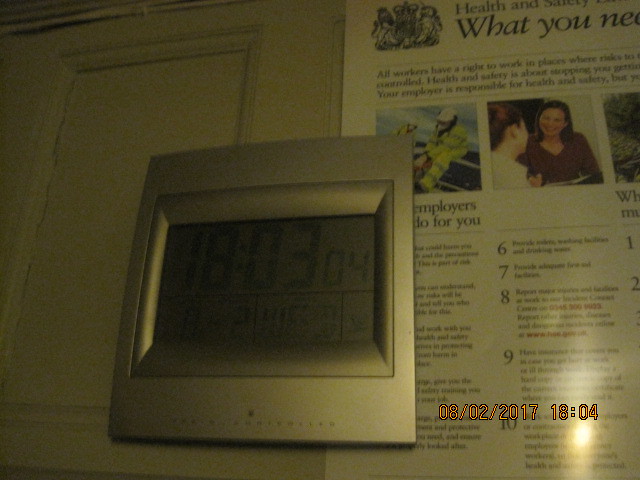This is an indoor color photograph, likely taken with a flash, depicting a digital thermostat affixed to a white-painted door featuring the typical four carved-out panels. The thermostat itself is set within a shiny gray panel and the digital LED display reads "1803" in a military-style format. The image is grainy and somewhat dark, obscuring some details, particularly on the lower half of the display. To the right of the thermostat, there is a laminated printout or newspaper article featuring numerous numbers and blocks of text that are largely unreadable due to the poor image quality. The lower right corner shows an overlay with the date "08/02/2017" and the time "18:04" in yellow text outlined in black.